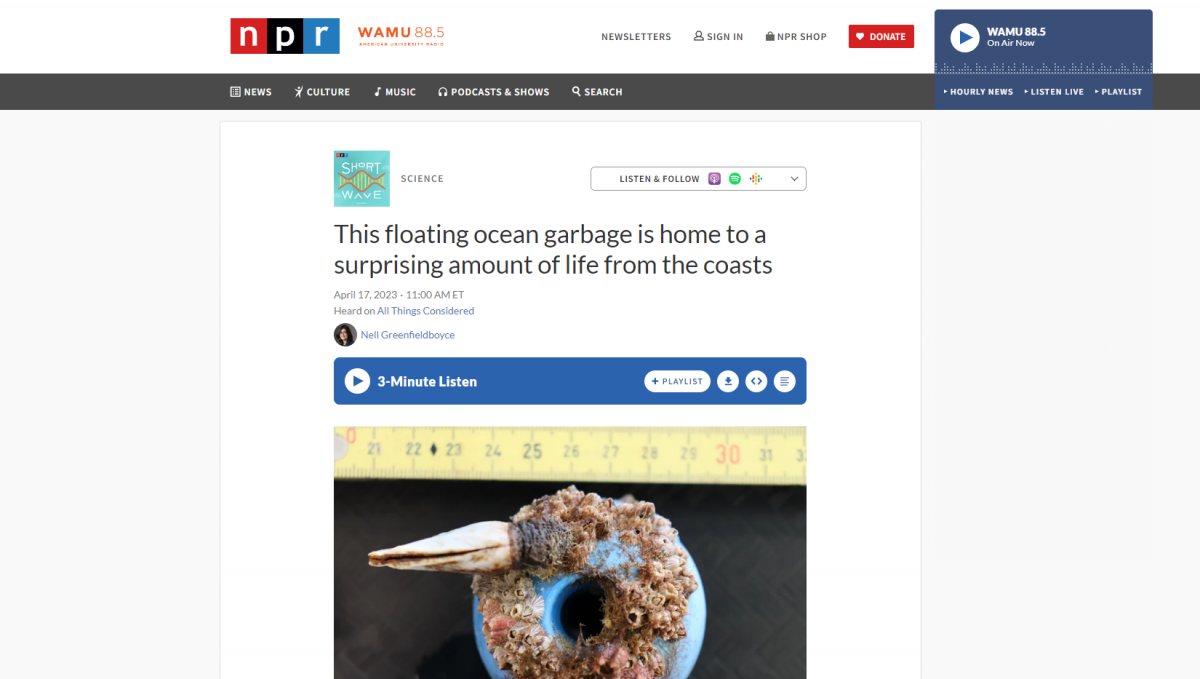The webpage features a clean white background with the prominent NPR logo on the upper left. The logo consists of white letters: 'N' in a red box, 'P' in a black box, and 'R' in a blue box. Adjacent to the logo, in red letters, reads "WAMU 88.5". Following this, from left to right, are links for "Newsletters," "Sign In," "NPR Shop," and a red "Donate" button. To the right of these, there's an icon to play a video and an additional "WAMU 88.5" label.

Below this top section, a black navigation banner lists options for "News," "Culture," "Music," "Podcasts," "Shows," and a "Search" bar. On the far right side of this banner, white text on a blue background provides links for "Hourly News," "System Line," and "Playlist."

Centrally positioned on the page is an image with the headline: "This floating ocean garbage is home to a surprising amount of life from the coast." Below this image is a profile picture of a woman, identified as Nil Green, with the name displayed in blue letters. To the right of this profile picture, a play button indicates a "Three Minute Listen" option, accompanied by a "Playlist" link.

Further down, another image showcases what appears to be a blue donut-like object covered in crustaceans, set against a black background. A tape measure is visible above the object, providing a sense of scale.